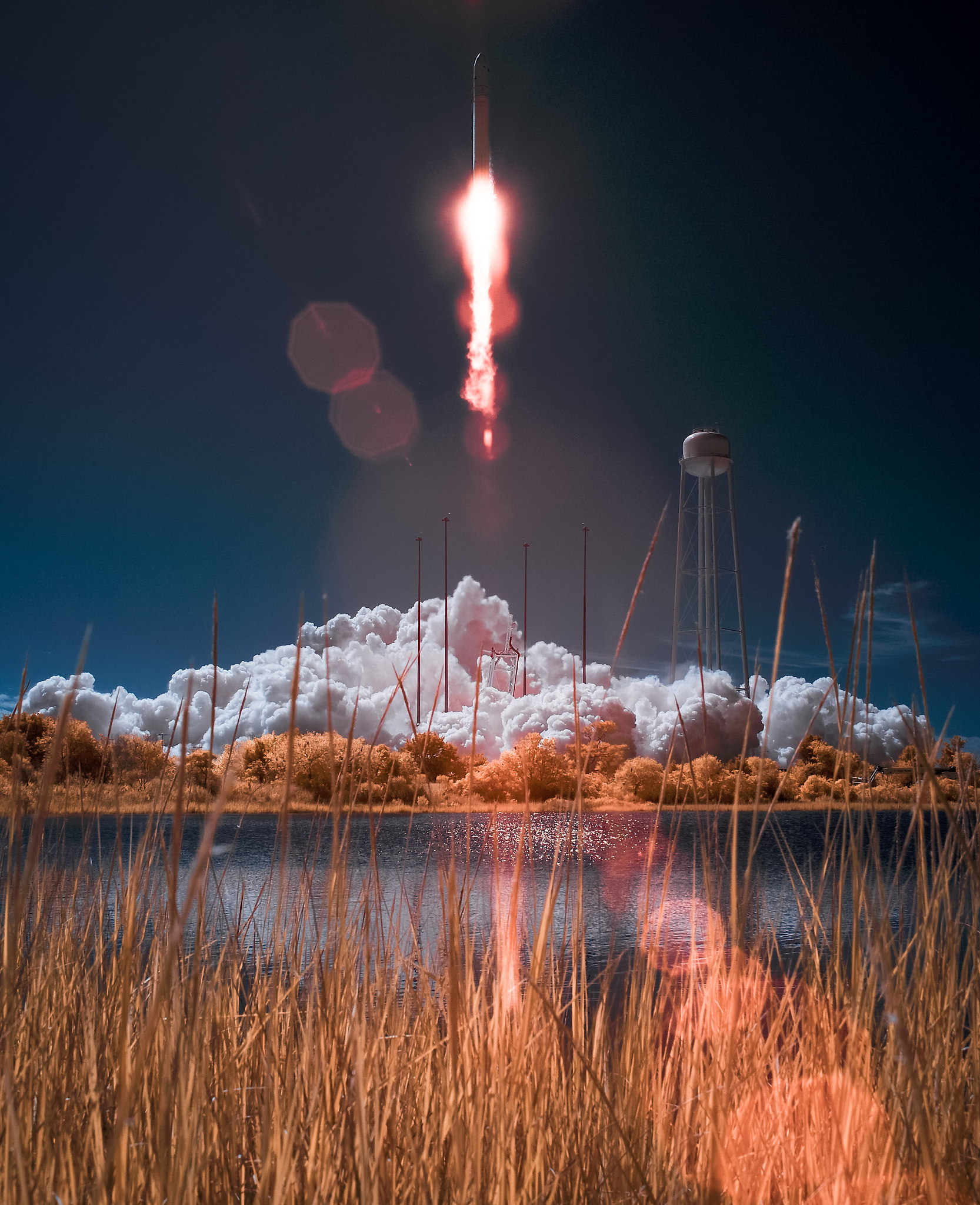This image captures a rocket launch taken from a low-angle perspective across a body of water. The rocket, perched at the center top of the photograph, ascends powerfully into a deep blue sky, with bright white and orange flames from its thrusters clearly visible. Beneath the rocket, a massive, thick white cloud forms from the condensation caused by the launch, spreading out dramatically along the ground. This cloud engulfs the base of a very tall, silver water tower situated on the right side of the image. 

In the mid-range, lining the edge of the shoreline, there is a row of golden-colored trees and brush, their shades reminiscent of dried grass or wheat, indicating a possible seasonal change. Matching this dried, golden hue, the foreground is filled with tall, dry grasses that extend across the scene, their tips reaching impressive heights, even higher than the rising smoke in some places. 

The surface of the water in the foreground reflects a soft white light, possibly lunar or from the rocket's own illumination, adding a gentle contrast to the otherwise dramatic scene. Lens flares trace diagonally from the upper left to the lower right, further enriching the striking visual elements of this photograph.